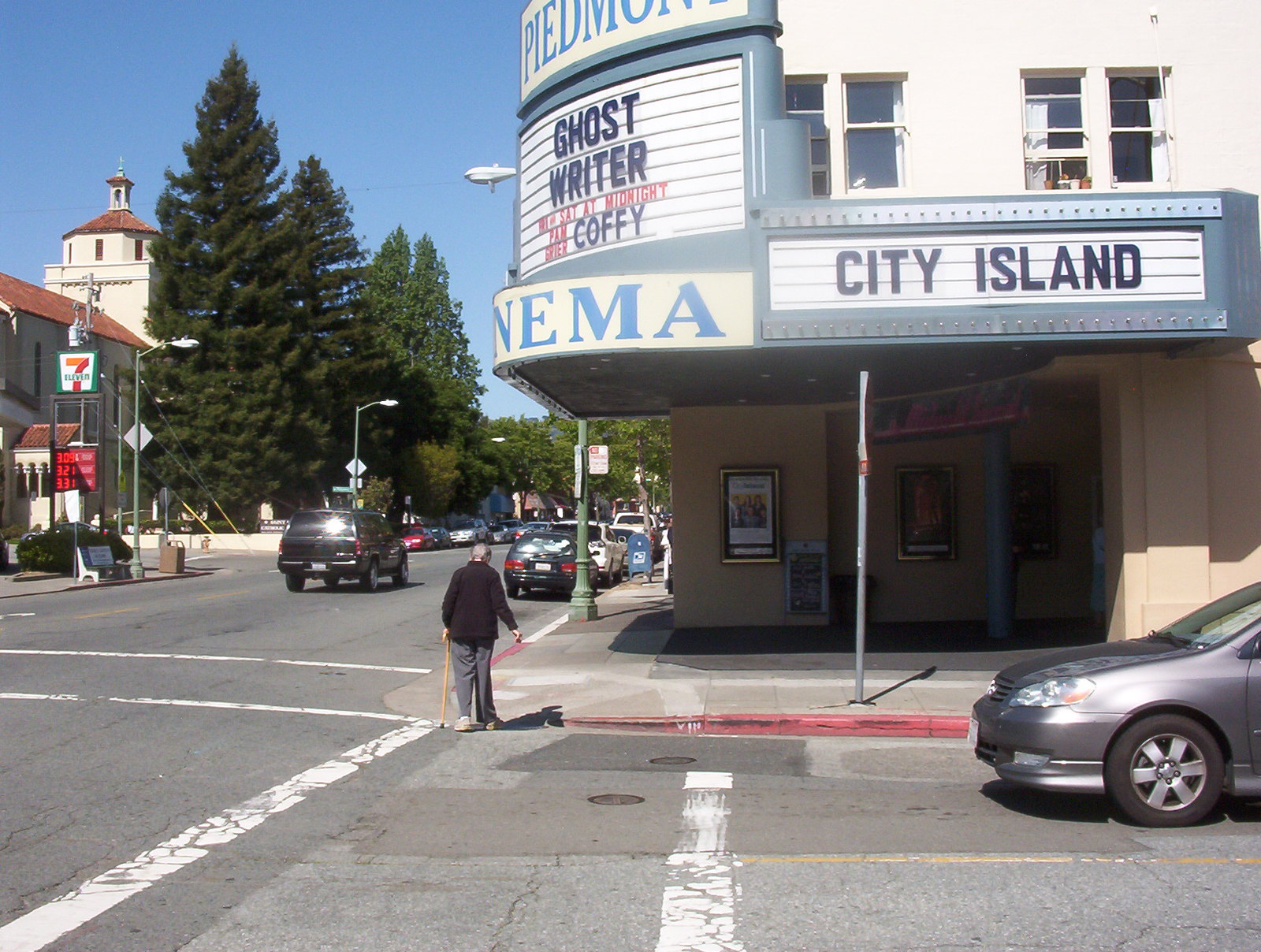This photograph captures a bustling city scene on a clear afternoon. Dominating the image is the Piedmont Cinema, an old-timey theater situated on the corner of a block with its curved facade. The theater's white marquee prominently displays "Ghostwriter" on the left side and "City Island" on the right. Beneath "Ghostwriter" in red letters, it announces a showing "Sat at Midnight," followed by "C-O-F-F-Y" in black. In front of the theater, an older person using a cane is stepping onto the sidewalk from a crosswalk, while a gray car is visible to the bottom right, stopped at the crosswalk. The upper left quadrant of the image features tall, thick conifer trees with a 7-Eleven store sign and gas prices visible below them. There is noticeable traffic, including parked cars on the left street and a black SUV driving by. The scene encapsulates a moment of urban life, framed by the charm of the historic cinema and the everyday hustle of city traffic.